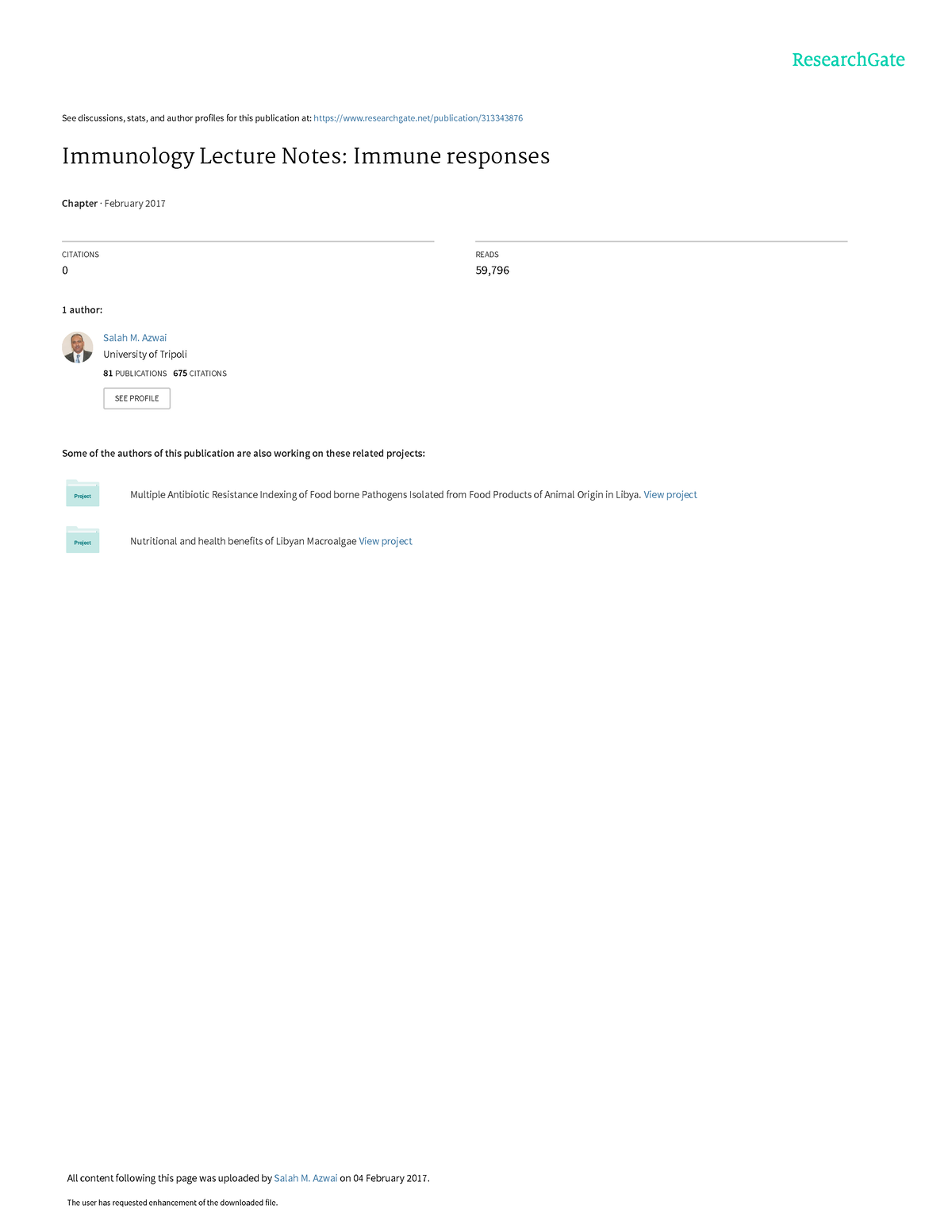This image is a screenshot featuring a white background, which seamlessly blends without clear boundaries. At the top-right corner, "ResearchGate" is prominently displayed in green. Below, in small black letters, is the phrase, "See discussions, stats, and author profiles for this publication at," followed by a blue, clickable link to "www.researchgate.net."

The main heading, "Immunology Lecture Notes: Immune Responses," appears in a larger font. Directly underneath, it states, "Chapter February 2017," with metrics indicating "Citation 0, Reads 59,796." 

A single author is listed, alongside a small profile picture of a man in a suit, blue tie, and white shirt. The author is "Salah M. Azoui" from the University of Tripoli, credited with "81 publications, 675 citations." There is also an option to "See Profile."

Further down, it notes, "Some of the authors of this publication are also working on these related projects," followed by two projects, each denoted by a green icon with the word "project" inside.

At the bottom of the page, there is a statement: "All content following this page was uploaded by Salah M. Azoui on February 4th, 2017."